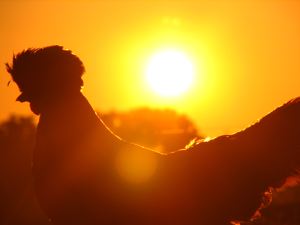This evocative image captures the silhouette of a rooster against a striking backdrop of the setting sun. The intensely bright sun sits low in the sky, a vivid white circle enveloped by a radiant yellow-orange halo that bathes the entire scene in warm hues. The sky itself transitions from light to deep orange, enhancing the dramatic contrast. In the foreground, the rooster stands with distinctive head feathers and a beak just barely discernible amidst its shadowy outline. Its tail feathers add a touch of texture to its form, but the overpowering brilliance of the sun obscures any intricate details or colors of the bird, reducing it to a majestic dark profile. The background features indistinct silhouettes, likely trees or vegetation, adding depth and composition to this artistic portrayal where light and shadow masterfully interplay.